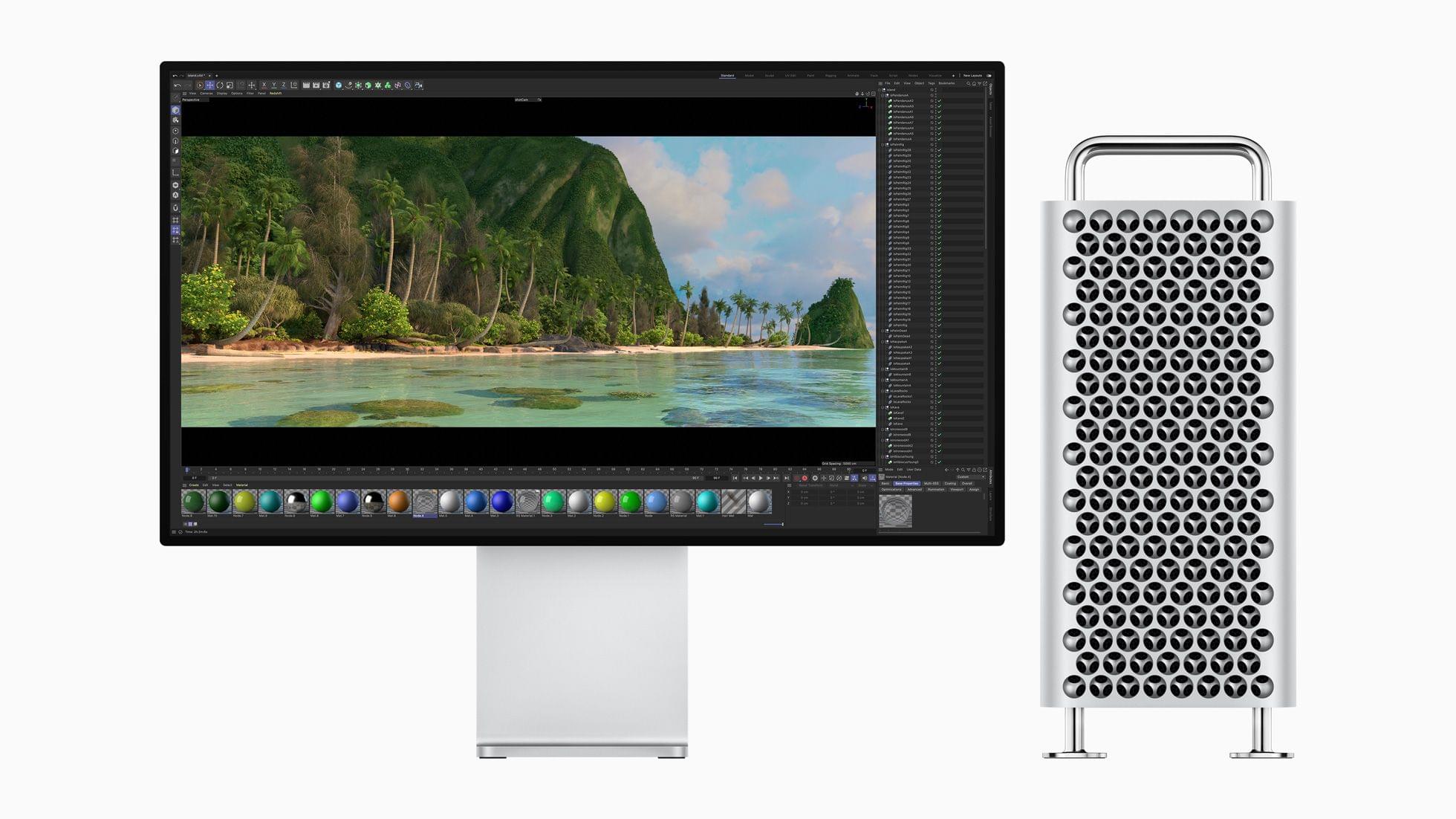In the center of the image, a black computer monitor is displayed against a white background. The screen shows a vivid island scene from the perspective of the water, which is a clear, light aqua blue, revealing green plant life beneath the surface. The beach is narrow, with about 15 feet of light brown sand, bordered by lush greenery, including trees, palm trees, and bushes. Towering above the beach is a prominent mountain with a green summit, framed by a medium blue sky dotted with white clouds. To the right of the monitor, there is a tall, rectangular piece of equipment resembling a stainless steel tower, possibly a computer tower or additional storage unit. This object has a perforated surface, similar to a cheese grater, and it stands on a silver metal stand. The overall composition suggests a clean, modern, and aesthetically pleasing scenario, possibly showcasing a workspace or a computer advertisement.